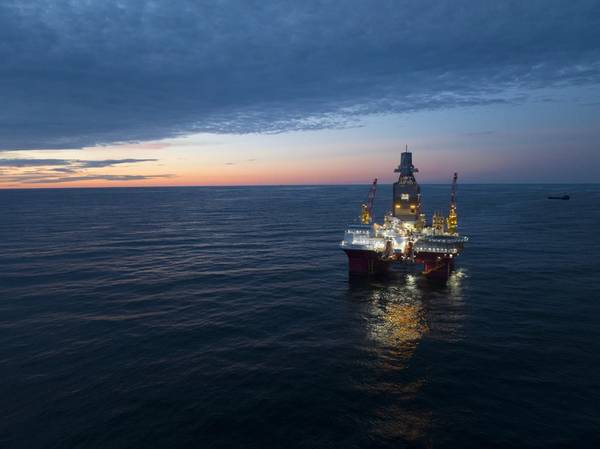This professional aerial photograph, taken over a calm ocean during a sunset, presents a striking scene where darkness softly envelops the surroundings, leaving just a hint of twilight. The sky, partially covered by dark clouds, bursts open at the horizon, revealing a golden glow that merges seamlessly with the tranquil, dark blue waters. The central focus of the image is an illuminated oil drilling platform or ship, equipped with towering cranes that cast a warm reflection upon the sea’s surface. The rig, featuring three towers with the middle one being the tallest, stands slightly skewed to the right, while a small boat lingers in the distant right background, adding depth and a subtle sense of movement to the composition.